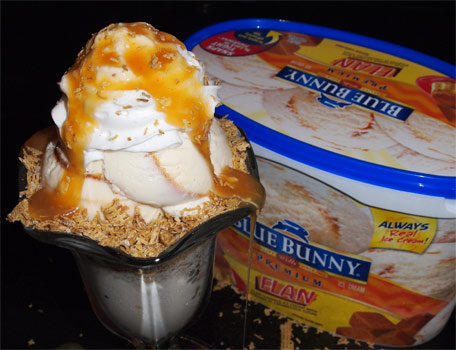In this image advertisement for Blue Bunny ice cream, a delectable homemade sundae steals the spotlight against a completely black backdrop. The sundae sits elegantly in a glass vessel, showcasing rich vanilla ice cream interspersed with caramel or butterscotch swirls. Topping off this creamy delight is a generous dollop of whipped cream, further adorned with caramel sauce that cascades down the sides of the sundae glass, creating a visually appealing drip effect. 

The ice cream itself appears to be garnished with a crunchy crumble, possibly resembling cereal or shredded toasted coconut, adding texture to the treat. Complementing the centerpiece, a Blue Bunny ice cream container is positioned to the right. This half-gallon tub features the brand's signature logo—a blue bunny in mid-leap—alongside labels emphasizing its premium quality and flan flavor. The packaging details include a blue and white text for the brand name and yellow-orange text boxes that read "premium" and "flan." The overall presentation not only highlights the deliciousness of the sundae but also underscores the quality and appeal of Blue Bunny’s ice cream.